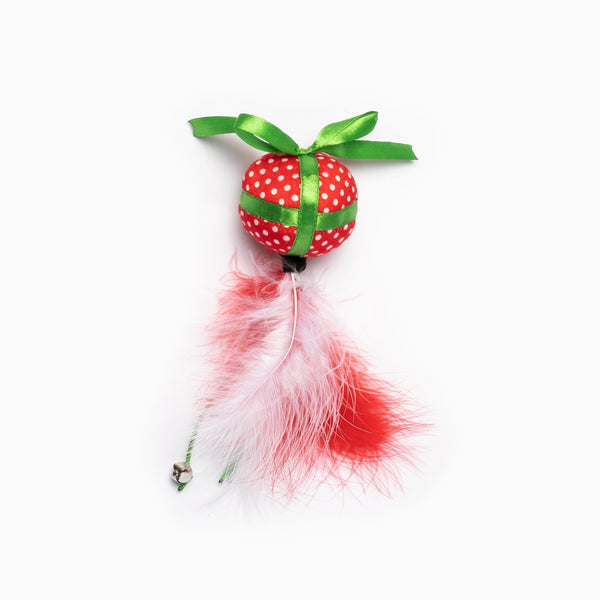This image features a festive ornament set against a mostly white background with a subtle grey tint. The centerpiece of the ornament is a red ball adorned with white polka dots, resembling the size of a bouncy ball or a strawberry. Wrapped around the ball is a shiny, satiny lime green ribbon that intersects both horizontally and vertically, culminating in a bow on top. Dangling from the bottom of the ball is a black bead, from which at least two feathers extend—one white and one red, though they blend together on the left side, making it seem as though there might be a third feather. Additionally, a small green tassel protrudes from beneath the bead, featuring a diminutive silver jingle bell at its tip. The ornament's vibrant red, white, and green colors give it a distinctly festive, Christmassy appearance.